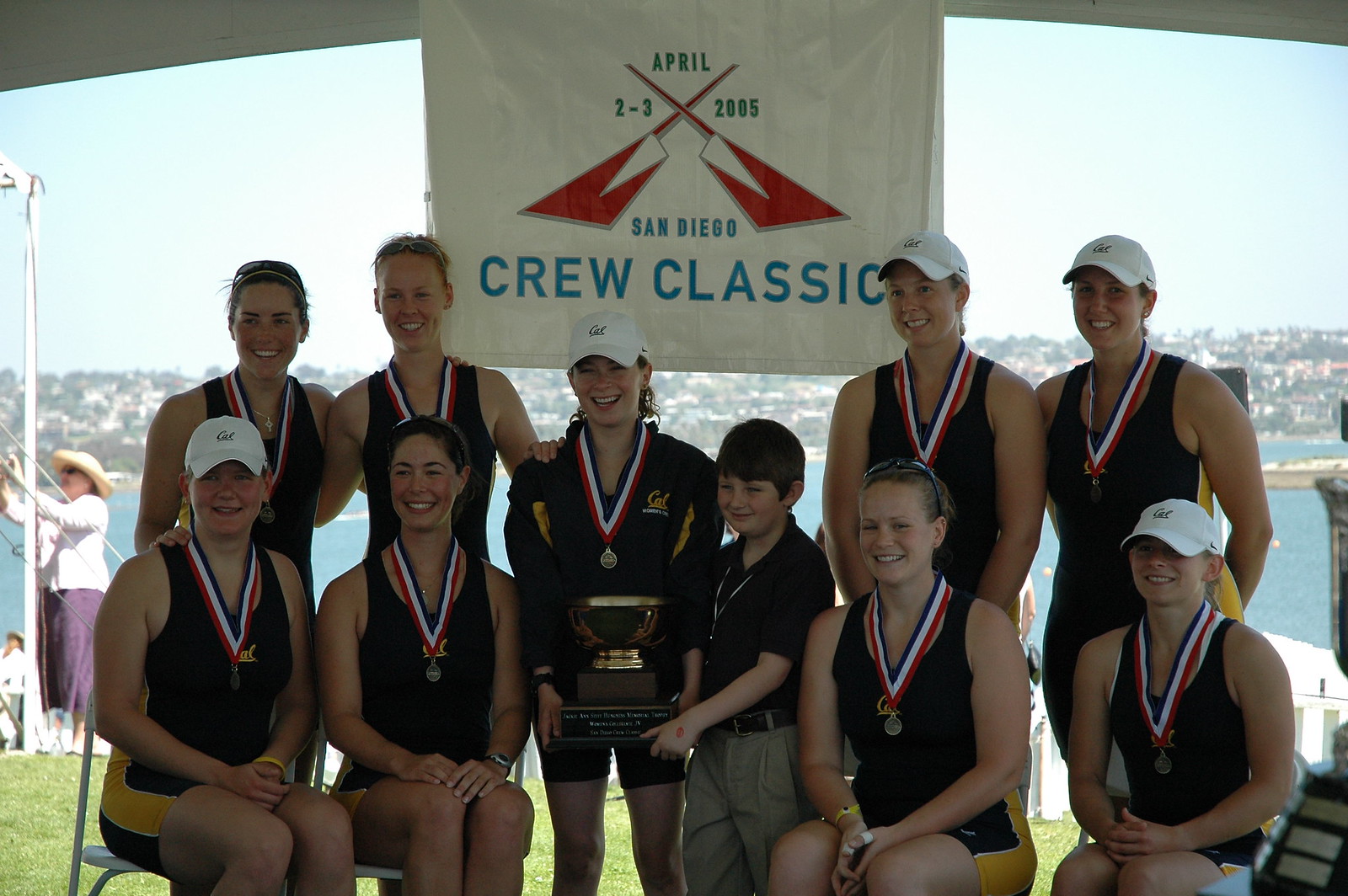This image captures a victorious moment of a crew team comprising mostly young women, likely between the ages of 18 and 20, with one very young boy, possibly around 7 or 8 years old. The group, who appears to have just completed a race, is posing outdoors against a picturesque backdrop of a harbor, flanked by homes, businesses, and trees visible across the water. They are gathered under a tent or canopy with a prominent white banner that reads, "April 2-3, 2005, San Diego Crew Classic," adorned with a logo featuring crossed white and red oars.

The team is arranged in two rows: four women are seated in the front row, and four more stand behind them, flanking the woman at the center who stands next to the young boy. Another woman stands slightly apart at the back. They are all dressed in tight-fitting black and yellow apparel—likely their team uniforms—accentuated by black and gold swimsuits. Most members sport white baseball-style caps, many of which bear the logo "Cal," indicating their affiliation with Cal University in California.

Each member wears a medal with a red, white, and blue ribbon around their neck, suggesting they've been awarded for their performance. The central woman and the young boy jointly hold a large, bowl-shaped trophy, signifying their team's accomplishment. Everyone is beaming with joy, capturing the essence of their triumph and the completion of their race.